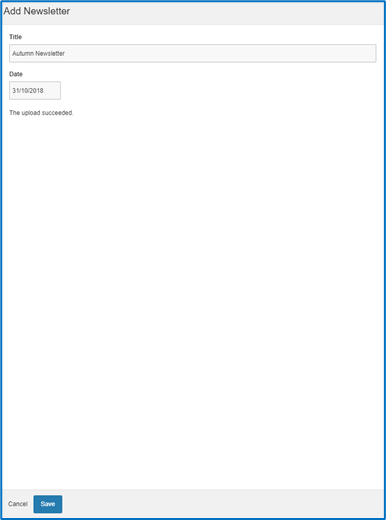**Detailed Caption:**

The image is a screenshot of an upload page, primarily displaying the top section. At the very top, there is a grey bar with the text "Add Newsletter" in black font. Below this bar, the main content of the page is set against a white background. The first visible field is labeled "Title" in black font, and the input field itself is grey with "Autumn Newsletter" written in black font inside it. Directly below the title field, there is a date field containing "31-10-2018," indicating October 31st, 2018, which is also Halloween. Further down, a message reads "Upload succeeded." All of this content is condensed into the top quarter of the page, leaving the remaining portion of the white background blank. 

At the bottom of the screenshot, there is another grey bar. On this bar, the word "Cancel" appears next to a blue button labeled "Save" in white font. The entire screenshot is bordered by a thin blue line, adding a distinct frame to the image.